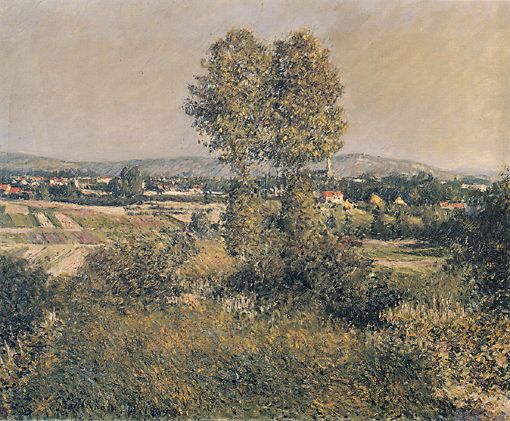This image portrays a detailed hand-painted landscape scene. In the foreground, dense foliage, including bushes, tall grass, and weeds, covers the terrain. Standing prominently in the midsection are two tall trees with intertwined branches. The image also depicts expansive farmland, plowed in characteristic shapes for crop cultivation. Scattered throughout the mid to background, there are old houses with reddish-orange roofs, which evoke the ambiance of a vineyard or a rural settlement. Beyond the farmland, hilly regions or small mountains rise gently against a sky that is somewhat cloudy but illuminated by sunlight, casting a bright glow on the grass and trees. The diverse palette includes shades of green, brown, yellow, tan, orange, pink, gray, white, and black, capturing the rich details and natural beauty of the outdoors on a sunny day.